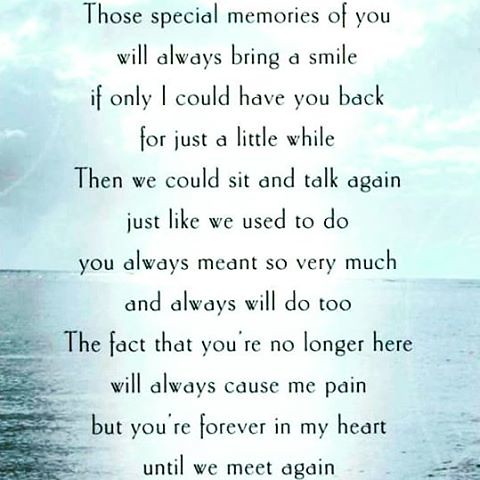The image appears to be a memorial or motivational card featuring a heartfelt poem. The background captures a serene ocean or river scene with the sun illuminating white clouds and reflecting on the water below, creating a peaceful ambiance. The text, which is centered both horizontally and vertically, is presented in a solemn font. It reads: "Those special moments of you always bring a smile; if only I could have you back just for a little while, then we could sit and talk again just like we used to do. You always meant so very much and always will do too. The fact that you are no longer here will always cause me pain, but you're forever in my heart until we meet again." The card conveys a sense of longing and fond remembrance, often associated with memorials or prayer cards for a loved one who has passed away.